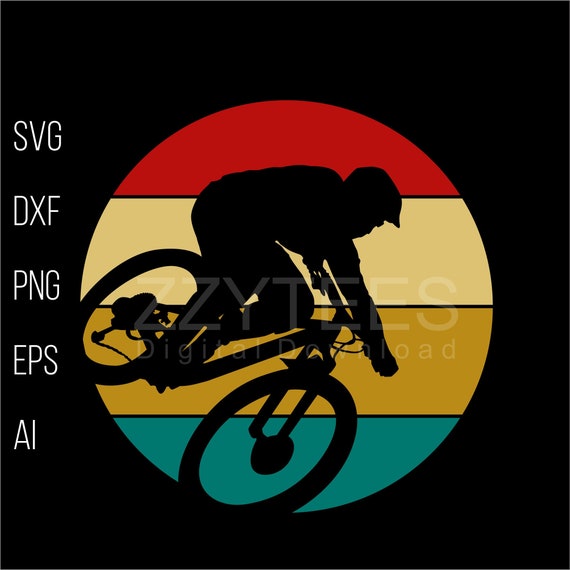The solid black background of the image features a prominent circular logo in the center, divided into four horizontal bars of vibrant colors: red at the top, a light tan (beige) below it, a darker gold middle section, and teal at the bottom. Inside the circle is a detailed silhouette of a person riding a mountain bike, appearing to be going downhill. On the left side of the image, in stark white font, is a vertical list of file formats: SVG, DXF, PNG, EPS, and AI. There are thin black lines separating each color strip within the circle. Additionally, a subtle watermark suggesting a digital download can be faintly seen on the image.